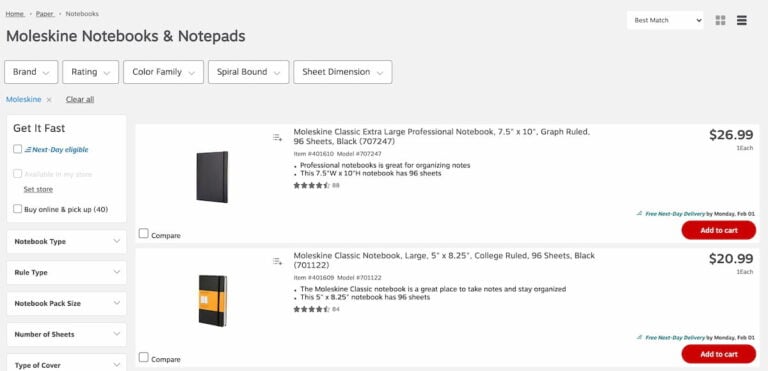The image depicts a detailed view of a website showcasing a selection of notebooks available for purchase. At the top of the webpage, navigation options are clearly labeled: "Home," "Paper," and "Notebooks." In the upper-right corner, there is a dropdown menu labeled "Best Match" for sorting options.

The website allows users to toggle between two viewing formats: a side-by-side view and a scroll-down view.

Beneath the navigation bar, several filtering options are available, allowing customers to refine their search by brand, rating, color, family, spiral binding, and sheet dimensions. The brand "Moleskine" is currently selected, with an "X" next to it for removal, and a "Clear All" option is accessible.

Further down, there are options under "Get It Fast" to select "Next Day Eligible" or "Available in My Store" with a "Set Store" function. Another checkbox option is available for "Buy Online and Pick Up," listing 40 items eligible for this service.

Additional filtering options let users specify preferences for notebook type, rule type, notebook pack size, number of sheets, and type of cover.

Two products are displayed prominently:

1. A black Moleskine Classic Extra Large Professional Notebook, measuring 7.5 inches by 10 inches, graph ruled with 96 sheets. The item number is (707247), priced at $26. It features options to compare via a checkbox at the bottom left and add to cart with a bright red "Add to Cart" button on the bottom right. It has garnered 4.5 stars from 88 ratings.

2. A Moleskine Classic Notebook Large, measuring 5 inches by 8.25 inches, college ruled with 96 sheets. The item number is (701122), similarly priced and equipped with a "Compare" checkbox and "Add to Cart" button. It shares the same rating of 4.5 stars from 84 ratings. 

Each product includes a thorough description, ensuring customers have all the necessary details to make informed purchasing decisions.